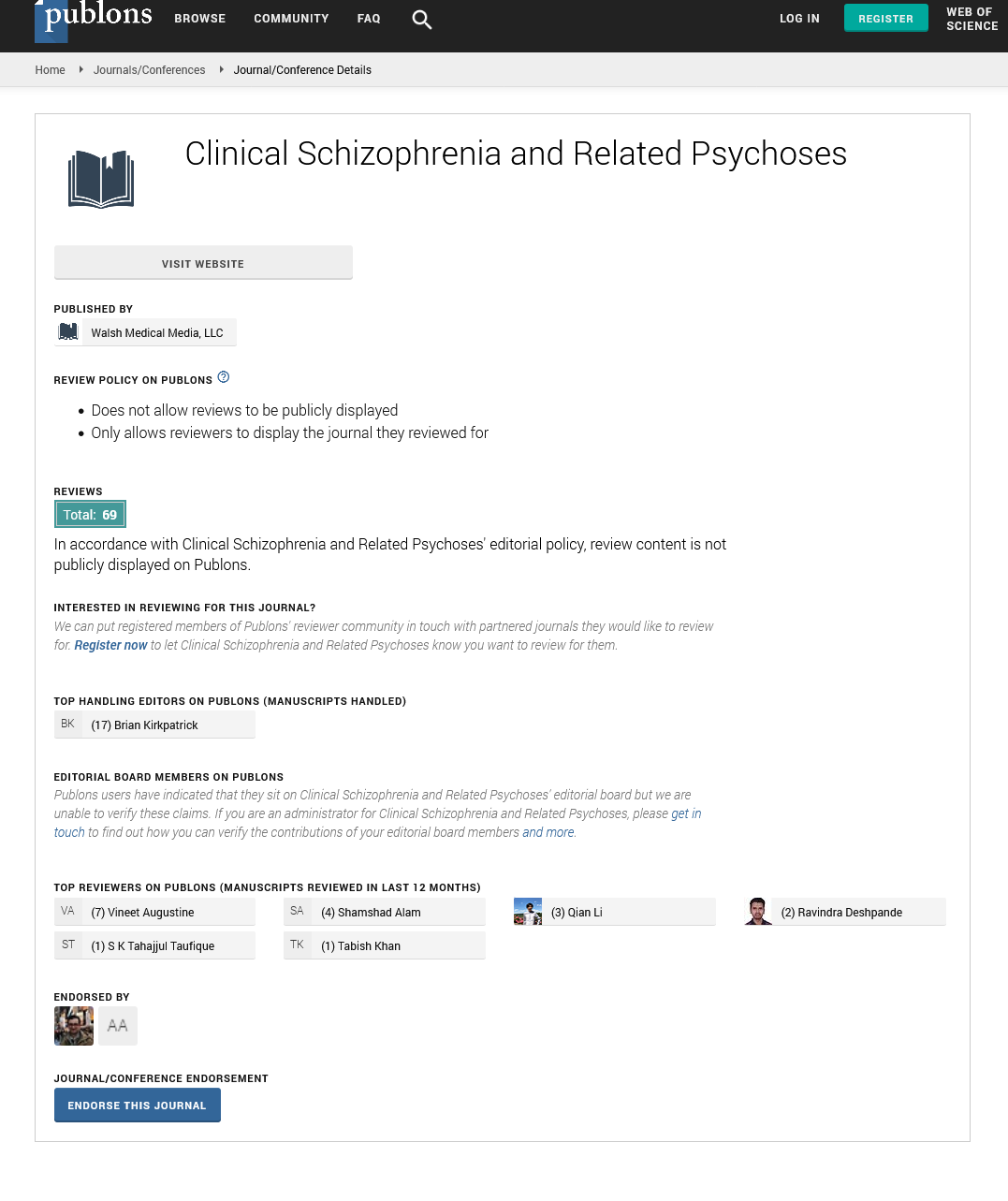Here is a detailed and cleaned-up descriptive caption for the image:

---

This image features a screenshot of a medical-related article from Publons, with the website name prominently displayed in the black-colored header at the top left corner. Alongside the website name, the header includes navigation tabs: "Browse in Community" and "FAQ," followed by a search bar, a "Login" link, and a green "Register" button on the right.

Beneath the header, a breadcrumb trail indicates the user's navigation path: Home > Journal Conferences > Journal Conference Details. The article is titled "Clinical Schizophrenia and Related Psychosis" and is accompanied by a graphic of an open book. Directly below the title, a "Visit Website" button is available, along with publication details indicating it was published by Welsh Medical Media, LLC.

The article has accumulated a total of 60 reviews, as noted by a green-tagged label. It also mentions that review content is not publicly displayed on Publons. Below this information, tags from top reviewers are shown, with several accompanied by picture avatars.

At the very bottom of the screenshot, there is a section labeled "Endorse By," indicating that two individuals on the platform have endorsed this article. In the bottom left corner, there is a blue "Endorse This Journal" button.

---